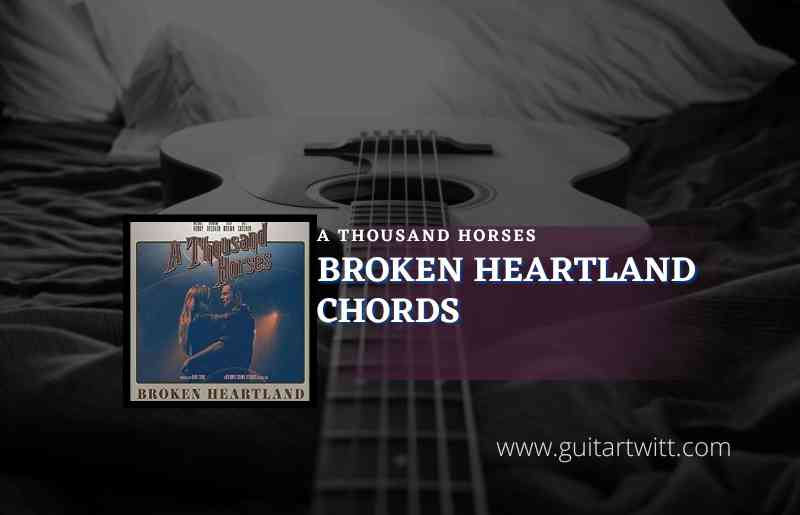The advertisement features a striking, darkened black and white photograph of an acoustic guitar, positioned such that the viewer is looking down the fretboard towards the guitar's body. The guitar rests on a bed with black crumpled fabric, while white pillows and fabric form the background. Superimposed on the left side of this image is the album cover for "A Thousand Horses Broken Heartland." This inset photograph showcases a dimly lit scene of a man and a woman embracing, bordered by a white frame. The top of the album cover bears the text "A Thousand Horses" while the bottom reads "Broken Heartland." To the right of the album cover, centrally located, the same text appears again: "A Thousand Horses" on the first line, "Broken Heartland" on the second line, and "Chords" on the third line, all in white font over a translucent purple bar. The image is a blend of color and monochrome elements, creating a somber yet vivid aesthetic, and is completed by the website www.guitartwit.com in white font in the bottom right corner.